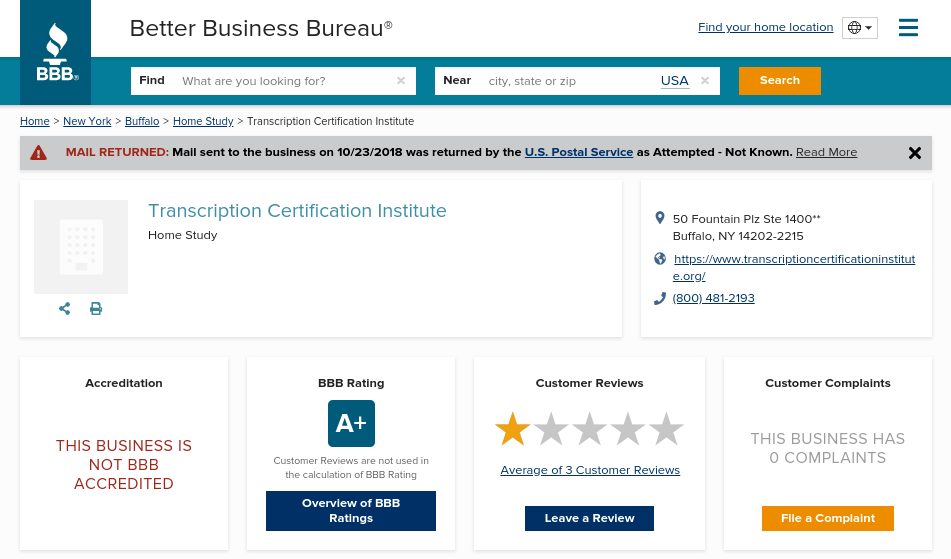**Detailed Description of the Screenshot from the Better Business Bureau's Website:**

The image captures a screenshot of the Better Business Bureau's (BBB) website. At the very top of the page, in black text on a white background, the words "Better Business Bureau" are prominently displayed. In the upper left corner, there's a blue rectangle featuring the white BBB logo.

On the top right, there is a clickable link in blue text that reads "Find your home location." Directly below this link is a search bar divided into two sections: the first box is labeled "Find, what are you looking for?" and the second is labeled "Near, city, state, zip." These input fields are followed by an orange search button on the right-hand side.

Beneath this search bar, the background remains white and includes several blue hyperlinked texts that say "Home," "New York," "Buffalo," and "Home Study." In black text, there is a link labeled "Transcription Certification Institute."

A gray banner immediately below these links contains a red triangle with an exclamation point inside it, accompanied by a bold red message that reads "Mail Returned." The banner continues with black text stating, "Mail sent to the business on 10-23-2018 was returned by the US Postal Service as attempted not known."

Further down, blue text reads "Transcription Certification Institute Home Study," followed by an address and the term "Accreditation." The subsequent section indicates that this business is "Not BBB accredited." Despite this, the business holds an "A+" rating. Additionally, customer reviews reveal an average rating of 1 out of 5 stars based on 3 reviews, and the business has zero complaints recorded.